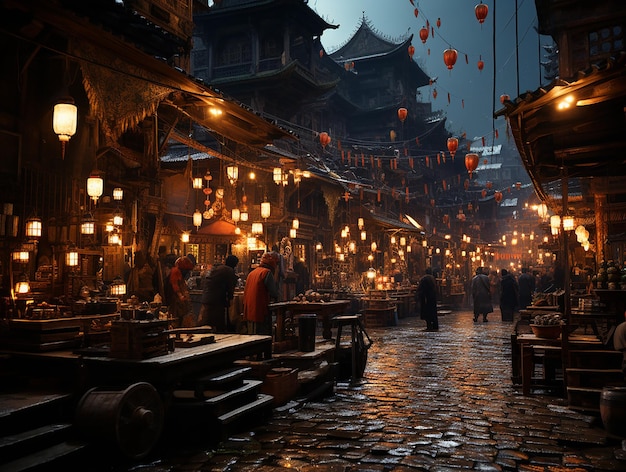The image depicts a lively nighttime street scene in a traditional East Asian district, possibly China or Japan, with rich details that blend a sense of cinematic or photographic quality. The composition is set within a rectangular frame where the longer sides are at the top and the bottom.

The street, paved with rectangular cobblestones, curves slightly to the right as it extends into the background. On either side, buildings made from tan-colored wood line the street, with the right side featuring at least two-story structures and the left side at least three-stories. The architecture displays traditional style with square or cubic shapes and rooftops that curve upwards into points or four-sided pyramids, characteristic of East Asia.

Stringed lanterns, hanging from informal lines running from left to right across the image, dominate the scene. These cylinder-shaped lanterns exude a warm beige light, complemented by small red flags and occasional round red lanterns. The cobblestone street is further illuminated by peach-colored lights that reflect off the surfaces of the buildings, which might also appear tan due to the lighting.

The lower right corner showcases a simple, minimalist wooden staircase and platform, while to the left, another small set of steps and an adjacent large wooden spool in dark brown occupy the scene. The left side is bustling with activity; small outdoor vendor areas with glowing lights beneath their awnings suggest a marketplace atmosphere.

Among the silhouettes of people crowding the street, some are seated at tables, while others are possibly browsing the vendor stalls. The figures are mostly dressed warmly, suggesting a cooler climate. In the lower part of the image, a person covered in a red cloth has their back partially to the viewer. 

Framing the vibrant street scene, lines with ropes and red flags arc slightly downwards between buildings. On the right side, a dark, boxy building features a grid window with nine panes on the top floor and an open patio area below, dotted with multi-colored pots containing plants. A second-floor balcony adorned with golden edges and columns adds to the intricate architectural details.

Overall, the scene is a harmonious blend of traditional architecture, warm inviting lights, and a bustling evening market atmosphere, capturing a moment rich in cultural ambiance and intricate details.